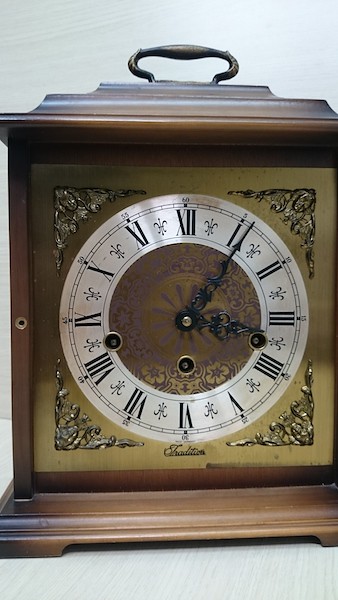The image showcases an antique-style decorative clock with a wooden housing and an ornate carrying handle at the top. The clock face is gold with numerals depicted in Latin figures, adorned with floral-patterned metal hands—one pointing toward the first numeral and the other just past the third. Fleur-de-lis embellishments grace the spaces between the numerals. Three gold rivets are positioned in the central circle, adding to the clock's intricate design. Thick gold borders accentuate the four corners of the outer square area, enhancing its elaborate appearance. At the bottom of the clock face, black cursive text can be seen. The wooden housing extends to the bottom of the clock, and the entire piece rests on a cream-white floor background.